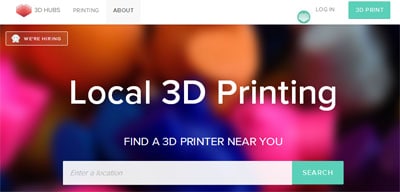The image showcases a vibrant web page header for a local 3D printing service. Dominating the center is the main heading, "3D Printing," with a subtitle below that reads "Find a 3D Printer Near You." A search bar, featuring a placeholder text "Enter location" and a green "Search" button, is positioned prominently on the right. To the upper right corner, there are two buttons: a "Login" button and a notable "3D" button. 

A striking "We're Hiring" banner with a bold red background occupies the top left corner, drawing attention to potential job opportunities. The background of the header is an out-of-focus, colorful blend of red, orange, and purple hues, possibly representing the diverse filament colors and the unlimited potential of 3D printing. This blurred backdrop effectively highlights the crisp, clear text, making the essential information stand out.

In summary, this header provides clear navigation options while also capturing the dynamic and creative nature of the 3D printing service. The visually appealing design and straightforward layout make it an inviting introduction for users interested in exploring local 3D printing options.